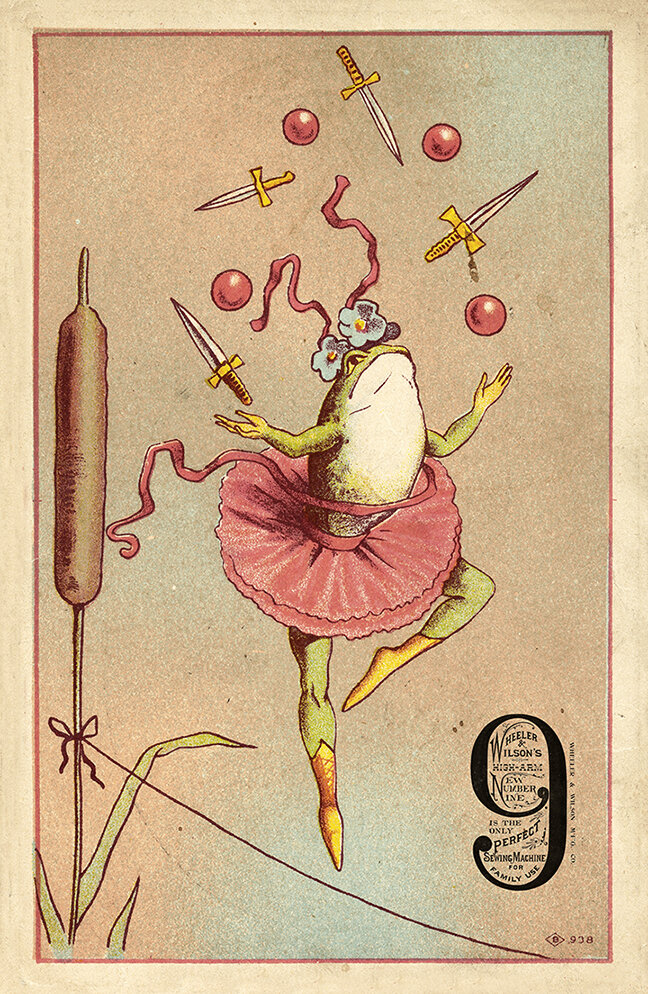This illustration depicts a whimsical scene featuring a frog performing an intricate balancing act. The frog, donning a pink ballerina tutu wrapped with a flowing ribbon and yellow ballerina shoes, confidently tightrope walks on a rope fastened to a cattail, which resembles a corndog. The frog, with green legs and a white torso, has blue petals adorning its head and juggles an array of objects including four red spherical balls with white reflections and four daggers with silver tips and yellow handles. The background showcases a light pinkish-brown hue with hints of blue, adding to the playful atmosphere. In the bottom right corner, there is a prominent number 9 logo, accompanied by text suggesting this might be an advertisement, possibly for a sewing machine described as "the only perfect sewing machine," lending a touch of vintage charm to the lively image.